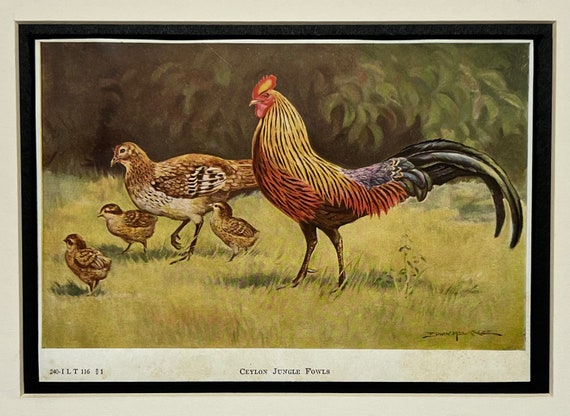A framed artwork depicting an old-style painting with a blend of brown and green tones. The horizontal-oriented frame is thin and light cream-colored, featuring a black matte border and a larger off-white border with text on the lower left, including "240 ILT 116." Centered in the image is a colorful rooster with yellow, red, blue, and black feathers standing on a patch of yellowish-brown grass. Accompanying the rooster are a female brown and white quail-like bird and three small brown chicks. Behind them, the backdrop consists of dark greenish-brown vegetation. The painting's title in the middle of the lower border reads "Ceylon Jungle Fowls," and a signature appears in the bottom right corner.